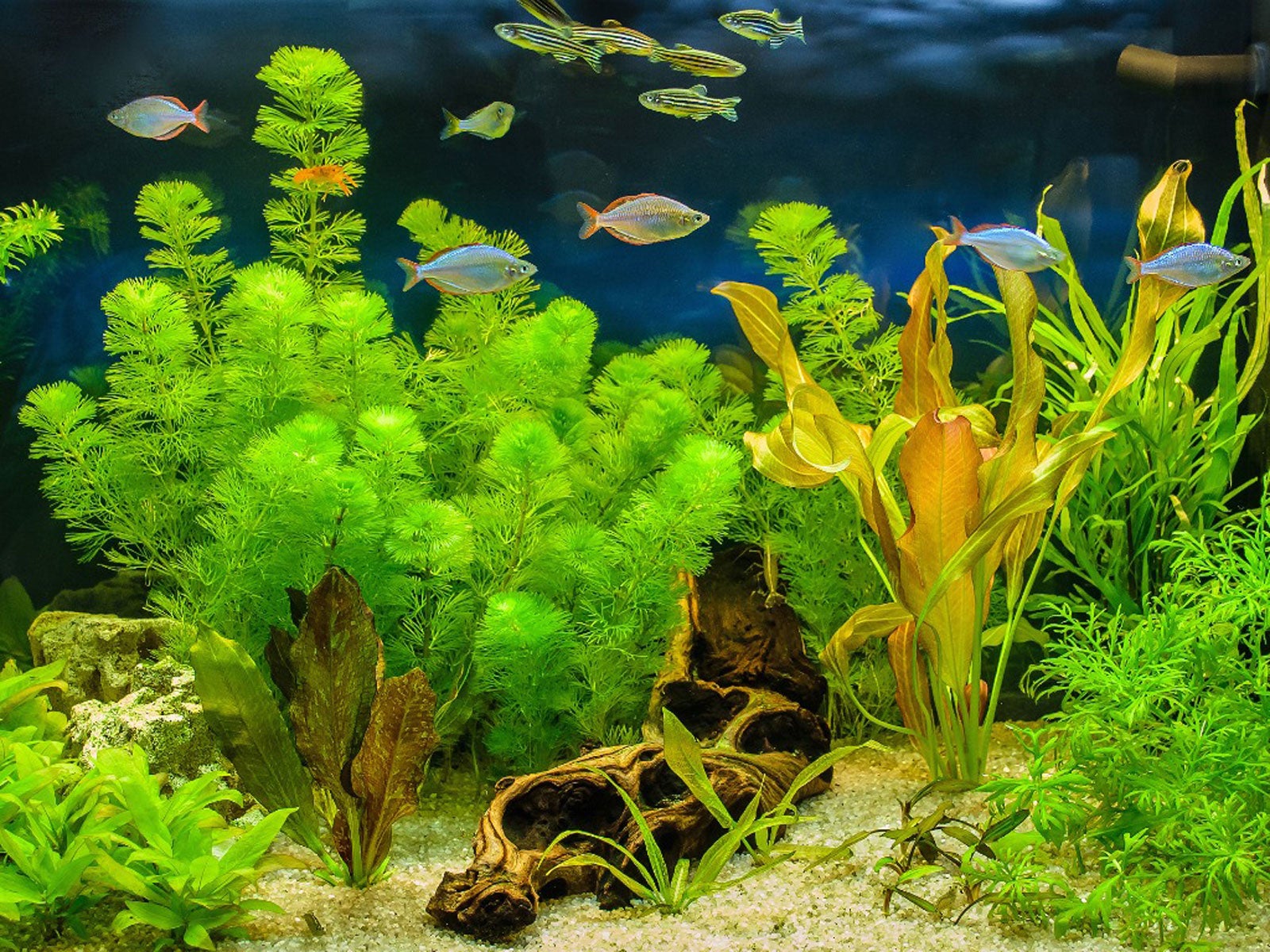The image depicts a vibrant underwater scene in a well-lit aquarium enclosure. The tank is abundant with vegetation, featuring a mix of real-looking plants and plastic or fake green and yellow foliage. A wooden log or decoration sits centrally amidst the greenery, anchored to a stone-covered ground. Numerous small fish swim throughout the clear water, including neon yellow and black striped fish, shiny red and blue fish, and clusters of orange and blue fish.  Some shrimp are also visible. The backdrop includes reflections of the fish against the glass, heightening the sense of depth. Near the upper right-hand corner, a pipe likely connected to the aquarium’s filtration system can be seen. The scene is lively and meticulously arranged, reflecting a carefully maintained aquatic environment.